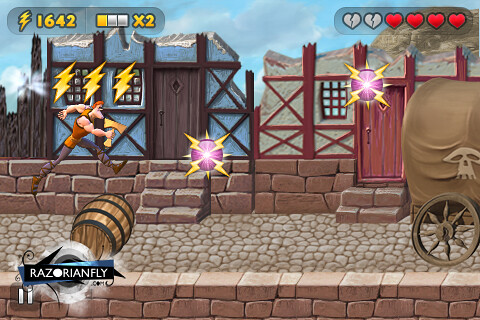A screenshot captures an intense moment from a video game in progress, showcasing a character's action-packed journey. The scene depicts a cartoonish, muscular man adorned in a sleeveless tunic and tall boots, leaping deftly over a large barrel on a cobblestone street. He moves horizontally from the left side of the screen towards the right. Ahead of the character lies a large covered wagon, adding an element of obstacle and intrigue to his path. Suspended in mid-air are two vibrant pink orbs emitting lightning bolts, with three additional lightning bolts hovering above the character, hinting at potential power-ups or hazards.

At the bottom of the screen, the name "Razor Ian Fly" is prominently displayed alongside a visible pause button, providing a moment of respite in the fast-paced game. The top left corner features vital game metrics: a score of 1642 accompanied by a lightning bolt icon, three "x2" multiplier boxes, and a life count indicating four out of six hearts remaining. This detailed snapshot not only captures the character’s dynamic motion but also offers a glimpse into the game's challenging and electrifying environment.